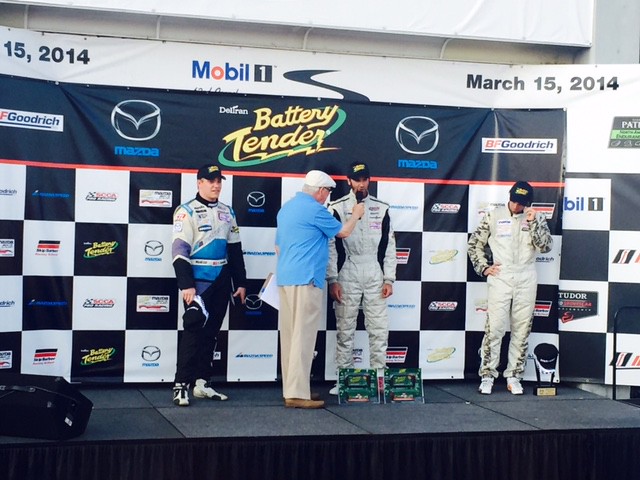In a photograph taken on a calm day, four men are standing on a black stage adorned with a large checkered backdrop showcasing various sponsors, including Mazda, Mobil, Goodrich, and Battery Tender. The focal point is the central figure, a racecar driver in a white racing uniform and black hat, being interviewed by an older man dressed in a blue shirt, white cap, and khaki pants, who is holding a microphone up to him. The backdrop behind them prominently features a banner that lists the sponsors and the date, March 15, 2014. Flanking the central racer are two other drivers; the one on the right also wears a white racing suit and black hat, while the man on the left dons a multi-colored tracksuit and black hat with the "Battery Tender" logo. Two square-shaped trophies are positioned at the feet of the central figure, adding to the celebratory atmosphere of the scene, which appears to be set at a champion’s podium following a race.